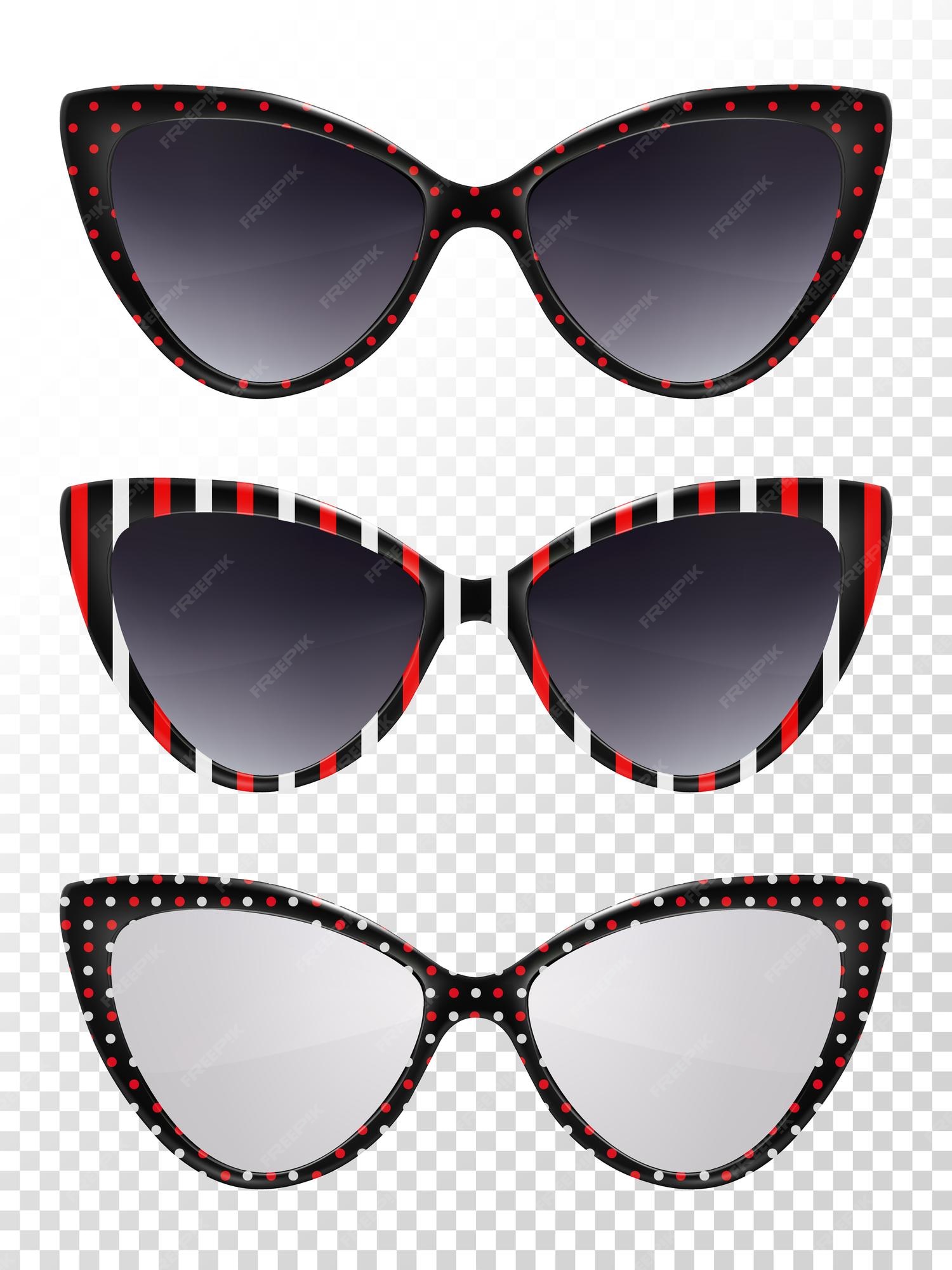The image features three digital art illustrations of retro-style cat eye sunglasses, set against a light gray and white checker pattern background, evocative of a transparent Photoshop layer. A white gradient spreads diagonally from the top left corner to about midway down the image. 

The top pair of sunglasses features black frames adorned with small red polka dots and dark gradient lenses that are concave, angling upwards into the corners. 

The middle pair maintains the cat eye shape but stands out with vertical red, black, and white stripes across the frame, transitioning into a black nose piece with a subtle white outline. These too are fitted with dark gradient lenses.

The bottom frames, also cat eye styled, are uniquely decorated with a multicolored grid of white and red polka dots over a black background, adding a playful and unusual flair to the collection.